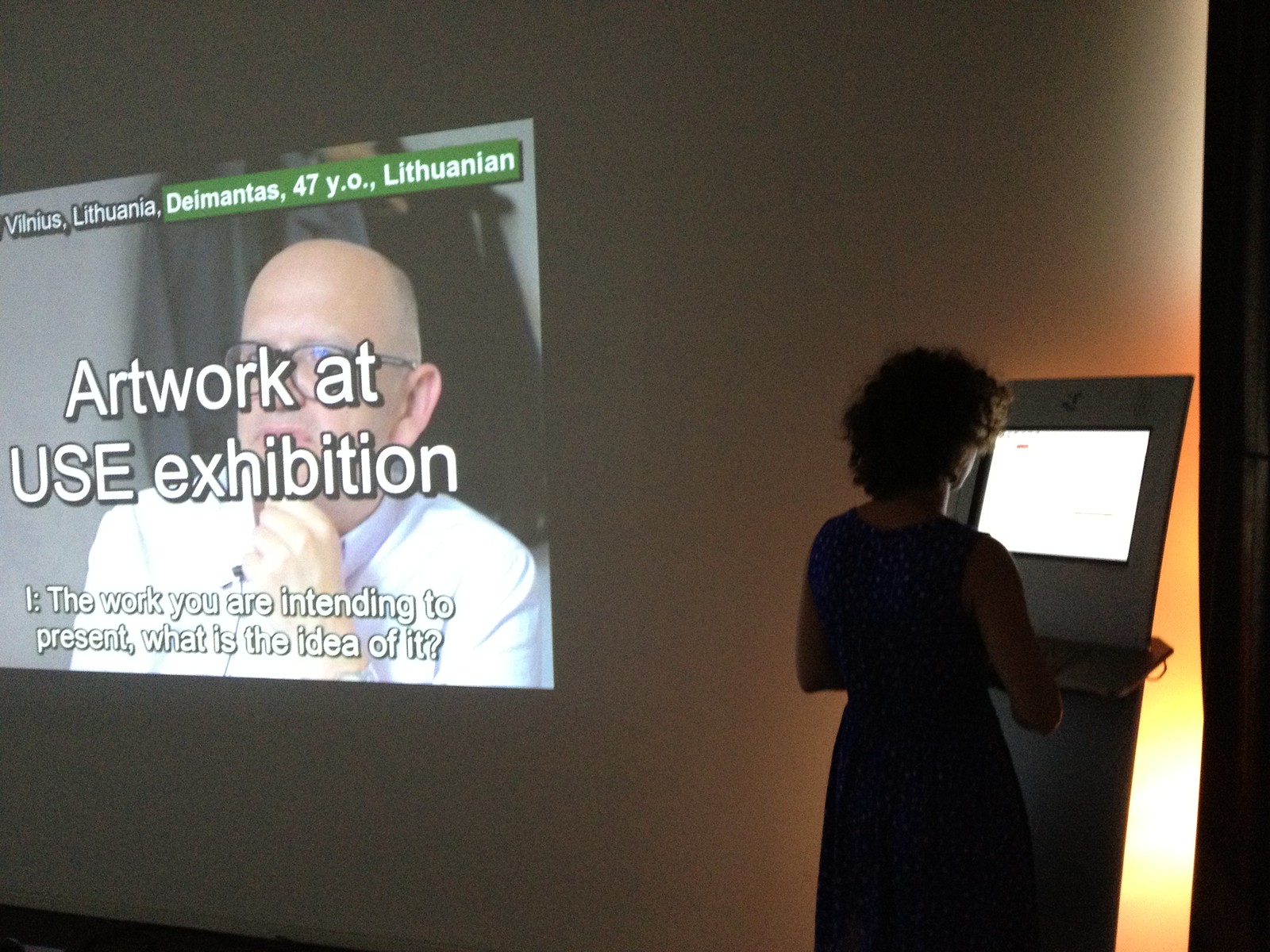This detailed color photograph captures a moment inside a dimly lit museum, showcasing a woman deeply engaged in an interactive art exhibit. The woman, positioned slightly to the right, stands with her back to the camera, focusing intently on a brightly lit small monitor. She sports short, curly brown hair and wears a blue dress. Adjacent to her, a stark white wall serves as a projection screen.

On this screen, a vivid image of a bald, middle-aged man is prominently displayed. The man, thought to be Deimontes, a 47-year-old Lithuanian, is depicted pensively with his left hand on his chin, wearing black glasses and a white shirt. Superimposed on his image are the words: "Artwork at U.S.E. Exhibition. The work you are intending to present, what is the idea of it?" Topping the projection, the text indicates the location of the event as "Vilnius, Lithuania."

The photograph effectively captures the contrast between the bright elements (the monitor and projection) and the otherwise dark room, emphasizing the silhouette of the woman at the interactive kiosk, immersed in viewing or interacting with the exhibit. The setup suggests a unique blend of digital art and viewer interaction, evocative of an immersive museum experience.